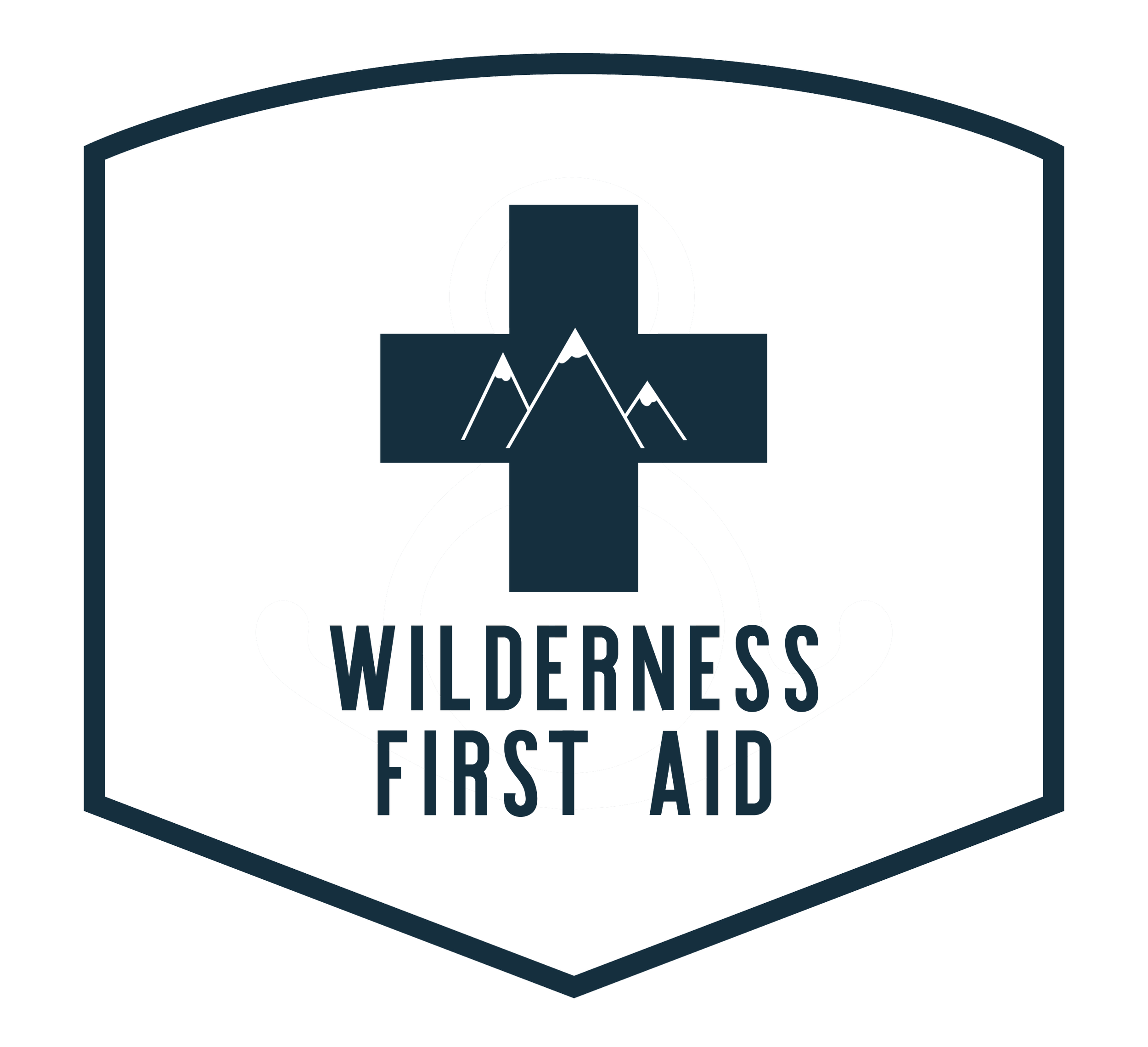The image is a logo for Wilderness First Aid, prominently featuring a distinctive design reminiscent of a Boy Scout patch. The emblem is uniquely shaped with a curved top and straight sides that taper down to a point, creating a half-diamond, half-square form. The border of the logo is outlined in navy blue. At the center of the white background is a navy blue cross, within which are three dainty, snow-capped mountain peaks, symbolized by triangles, adding an element of nature and adventure to the design. Below the cross, in capital letters, are the words "WILDERNESS FIRST AID," also in navy blue, offering a cohesive and clean visual appeal. The overall layout is meticulously organized, with a coordinated color scheme of navy blue and white, making it a striking and memorable logo that could easily be seen on a trail sign, certification patch, or uniform.